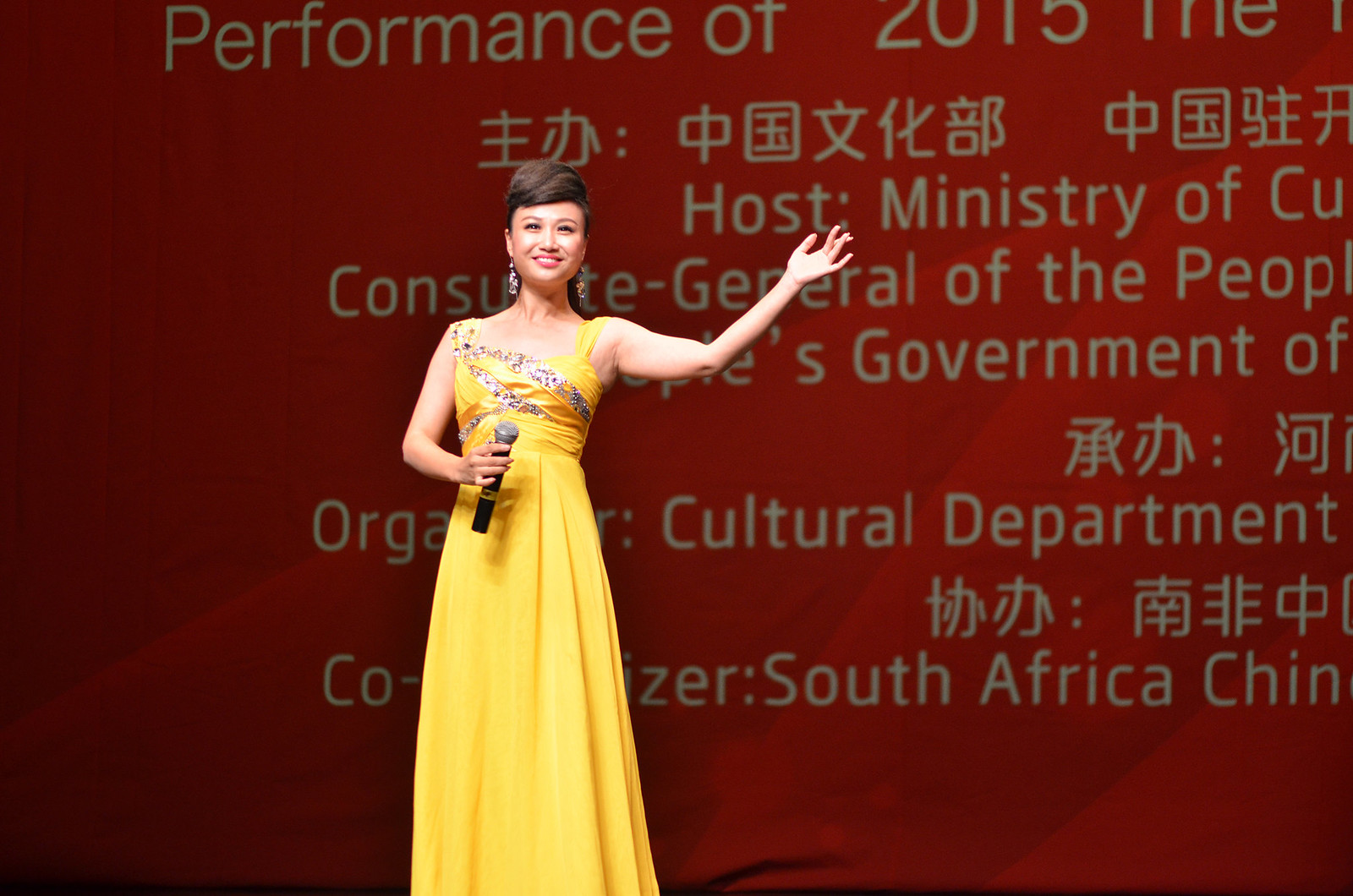An Asian woman is standing on stage, acknowledging the audience with a warm smile. Her hair is styled in a unique mohawk-like dome shape, short on the sides and swept over the top. She is wearing a striking yellow dress adorned with sparkling silver straps that cross her chest and waist, and she accessorizes with dangling, diamond-like earrings. She holds a black microphone in her right hand while extending her left arm in a gesture of gratitude or presentation. Behind her, a large projection screen displays white text over a deep red background, partially reading "Performance of 2015, the" followed by some Chinese characters. Below that, it says "Host: Ministry of" before cutting off, with additional partially readable text about organizers: "constitute general of the people, organizer cultural department," and "co-organizer South Africa, China." The woman appears to be highlighting or introducing the event, creating an engaging and elegant atmosphere.